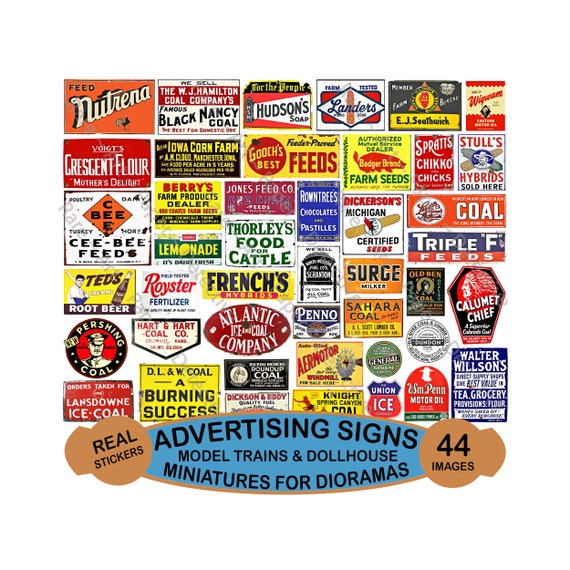This image showcases a collection of vintage clip art stickers intended for advertising signs, model trains, and dollhouse miniatures for dioramas. At the bottom, a brown oval shape features the words "Real Stickers" on one side and "44 Images" on the other, connected by a blue section with black text that reads "Advertising Signs, Model Trains, and Dollhouse Miniatures for Dioramas." Above this section, a variety of small vintage labels and logos are displayed in vibrant colors such as blues, yellows, reds, and oranges. Among these, notable labels include "Feed the Retrino with a Little Chicken," "W.J. Hamilton Coal Company's Black Nancy Coal," "Hudson Soap," "Landers," "E.J. Southwick," "Ted's Root Beer," and others dedicated to food, cattle feeds, fertilizers, and coal companies. The collection serves as a prototype to promote the sale of these clip art stickers for use in detailed miniature displays.